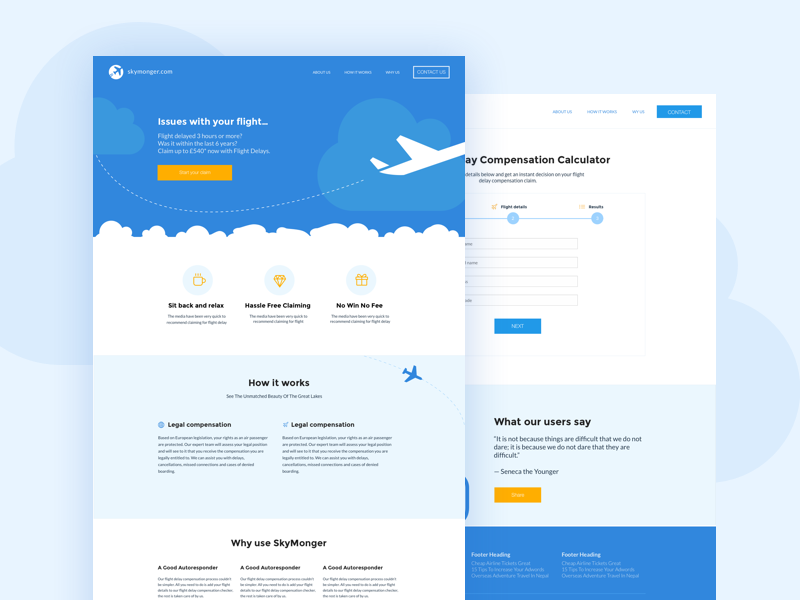This screenshot displays a dual webpage overlay against a pale blue background adorned with two iconic blue clouds—one positioned in the top left corner and the other in the bottom right. The right-side webpage is slightly lower, leaving some negative space above it, while the left-side webpage overlays about half of the bottom one and sits higher up.

Focusing on the top-left webpage, it features a blue header. In the header's top-left corner, there's a white circle containing a blue airplane icon angled at 45 degrees upwards to the right. Adjacent to this icon, the white text reads "Skymonger.com." On the top-right corner of this page, blurred white text makes up the first three sections, followed by a prominently displayed white box with all-caps text reading "CONTACT US." 

Below the header, the blue background is embellished with two cartoonish, lighter blue clouds—one partially visible on the left and another with just its right corner cut off on the right. Large white text near the top left states, "Issues with your flight..." Beneath this, three lines of smaller white text inquire, "Flight delayed 3 hours or more? Was it within the last 6 years? Claim up to 540 pounds* now with flight delays."

At the bottom of this section is an orange rectangular button with white text on it.